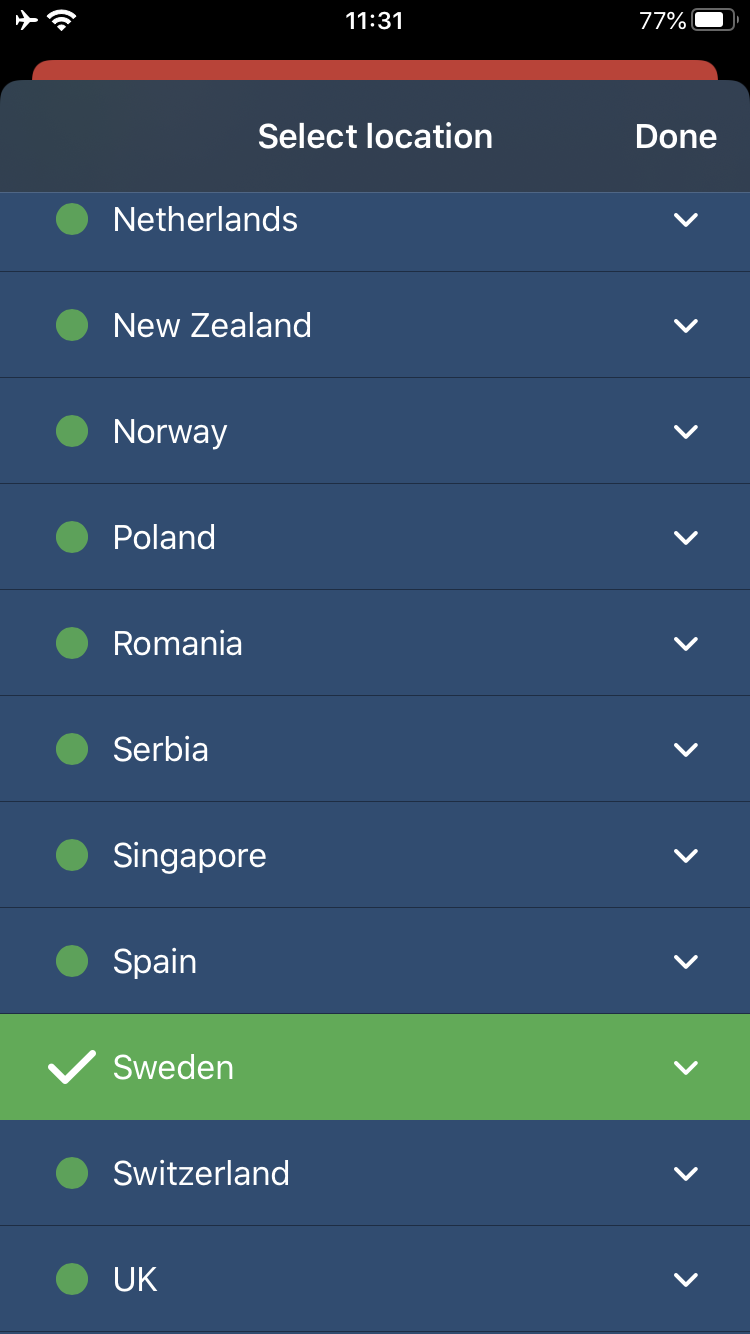"Screenshot of a Mobile Application Settings Page 

The screenshot captures a settings page from a mobile application with a sleek, modern design. The top section features a black header containing white icons centralized for easy visibility. Among these icons, a small white airplane icon and a Wi-Fi signal indicator (depicted with three rounded bars) are located on the top-left. On the top-right, it displays the battery life at 77%, represented both numerically and graphically with a horizontal white battery icon. The current time, 11:31, is displayed in white text, centered below the icons. 

Directly beneath the header, there is a small red rectangle with rounded top corners, followed by a slightly taller bluish-gray rectangle with similarly rounded top corners. This rectangle serves as a control panel with the text "Select Location" in white, centered and prominent, indicating that users can select locations. To the right of this text is a clickable 'Done' option.

Below this section, the interface transitions into a dark blue background where a list of country locations is displayed, separated by thin black lines. Each location entry consists of a white arrow pointing downwards on the right side and a green circle on the left, except for the selected location. To the right of the green circles, white text lists the countries in the following order: Netherlands, New Zealand, Norway, Poland, Romania, Serbia, Singapore, Spain, Sweden, Switzerland, and UK.

Notably, Sweden is the selected location, distinguished by a green background instead of the dark blue and a white checkmark replacing the green circle. This clearly marks the user's current selection.

This detailed description provides a comprehensive view of the settings page, enabling easy navigation and understanding of the functionalities."